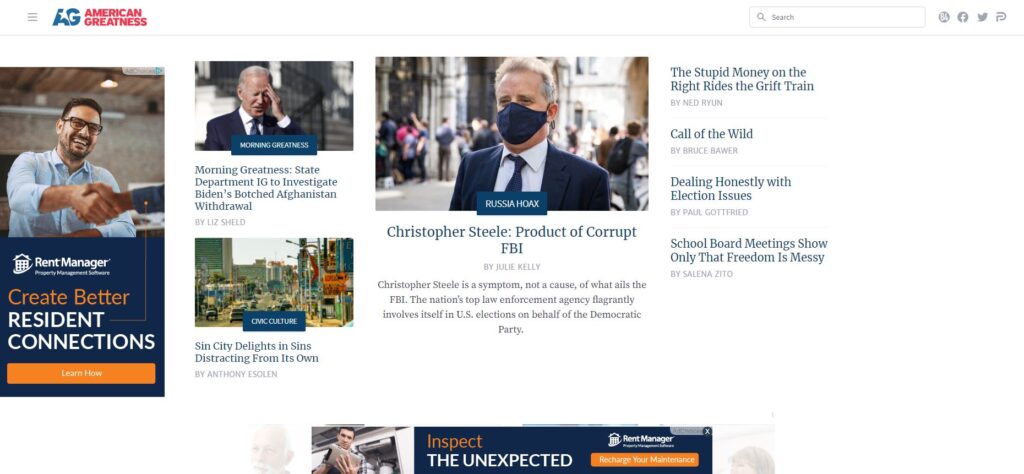This is a detailed description of a screenshot captured from a website on a PC or laptop. The website in question is "American Greatness," identifiable by its logo featuring a blue capital letter "A" slightly overlapping a "G," with the "A" adorned by a partial white star at the top. The masthead displays "AMERICAN GREATNESS" in bold red uppercase letters next to the logo. 

On the far right side of the screen, there's a search box accompanied by clickable social media links, including but not limited to Facebook and Twitter, located at the top right corner.

The most prominent post on the page is about Christopher Steele, described with the headline "Product of Corrupt FBI" and "Russia Hoax, Russia Hoax." The accompanying image shows a man with grey hair, likely Caucasian, wearing a mask (either blue or black) that covers his nose. He is dressed in a navy blue suit, matching tie, and a white collared shirt.

To the left of this post is an article titled "Morning Greatness: State Department, IG to Investigate Biden's Botched Afghanistan Withdrawal," illustrated with a photo of President Joe Biden. In the image, Biden is raising his hand to his forehead, positioning it just above his left eye.

Another article on the page is titled "Sin City Delights in Sins Distracting from its Own" under the category Civic Culture. Additionally, there is an advertisement on the far left for "Rent Manager" with the slogan "Create Better Resident Connections."

On the far right, a list of articles includes headlines like "The Stupid Money" and "Right Show Only That Freedom is Messy" by Selena Zito. These article titles are in light grey, with the author names making them somewhat challenging to read clearly.